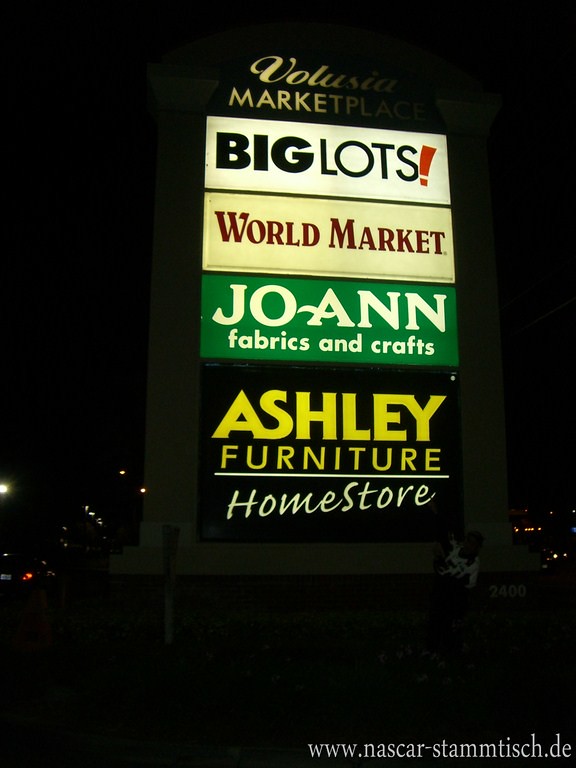The image captures a large, illuminated outdoor sign typically placed in front of a shopping department or mall complex. At the top of the sign, the text "Felucia Marketplace" can be faintly read, suggesting this is the name of the commercial area. The sign lists several prominent stores: "World Market", "Joanne Fabrics and Crafts", and "Ashley Furniture Home Store", from top to bottom. A person is faintly visible sitting beneath the sign, but the image is taken at night, making it difficult to discern details. In the bottom right corner of the image, a web address is partially visible, reading "www.nascar-stamtish.de", indicating a possible connection to a German-language website.